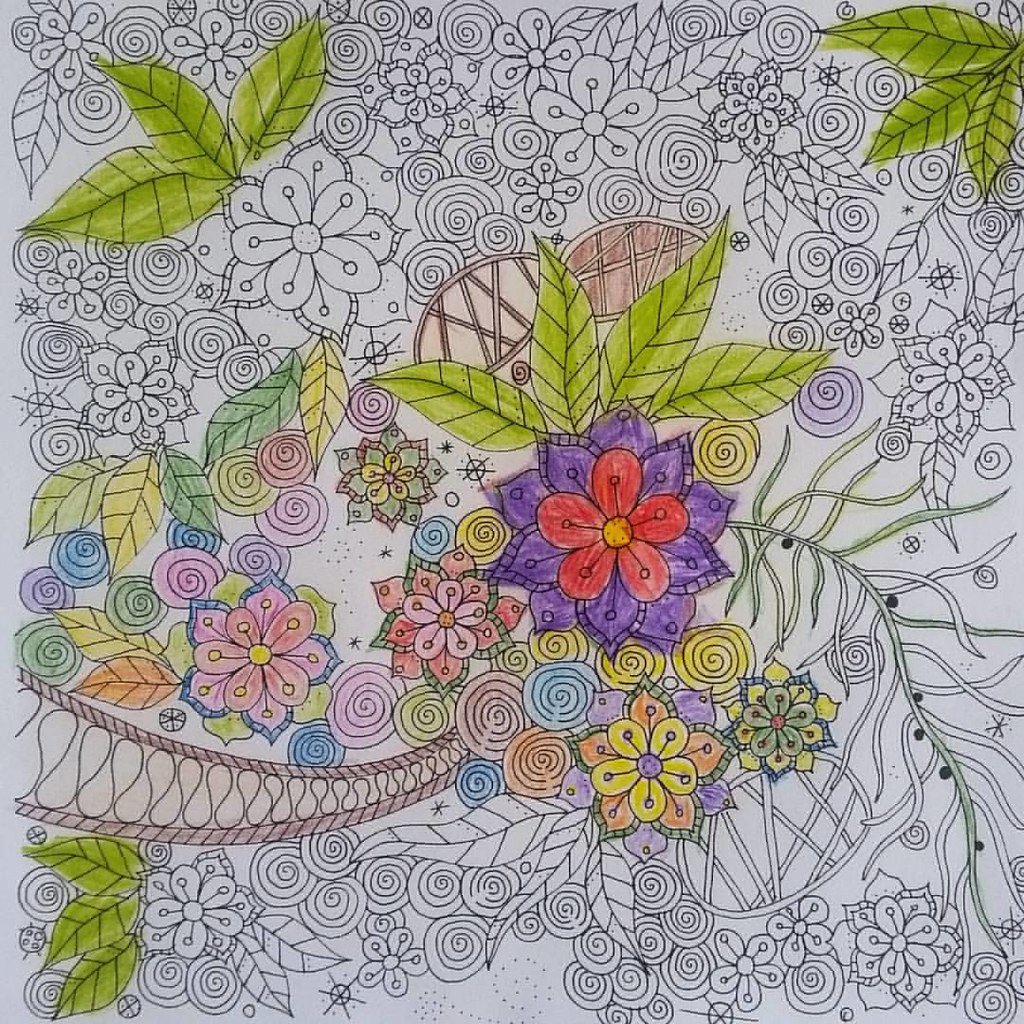This image depicts a partially colored page from an adult coloring book, showcasing a vibrant mix of flowers, foliage, and intricate patterns. At the heart of the composition is a striking flower with red inner petals and purple outer petals, centered around a yellow core. The artist has used a combination of colored pencils, and possibly crayon or watercolor, to bring this floral centerpiece to life, with some coloring noticeably extending beyond the lines. The surrounding leaves have been shaded in various green hues, contributing to the lively and detailed nature of the piece. Other flowers in the scene are tinted with pinks, and dynamic designs resembling swirling ribbons and circular spirals add to the complexity. The artwork is about one-third to slightly over one-third complete, highlighting the artist's ongoing journey in filling this elaborate page with color.